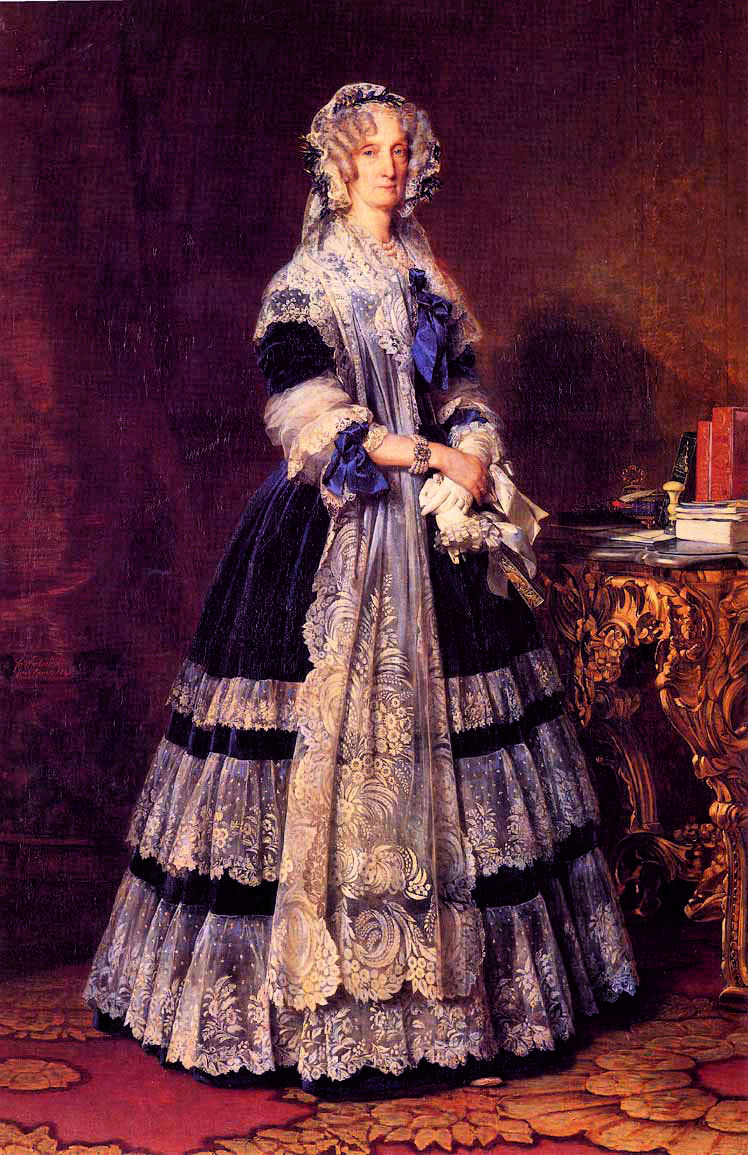This painting is a tall, rectangular, full-length portrait of a middle-aged woman dressed in an elegant, dark blue velvet and white lace gown. She stands at the center, gazing directly forward, her figure stretching from head to toe. Her attire includes a lacy shawl that drapes gracefully almost to the floor and a white upper-length glove on one hand. The gown is notably detailed with multiple layers of a lacy skirt. A delicate bracelet and pearl jewelry adorn her wrist and neck, while a blue and white lace bonnet sits atop her ringlet-curled gray hair. 

The background features a wall shaded in deep plum that transitions to burnt orange, providing a rich contrast to the woman's attire. Below her, a carpet with large, orange and yellow flowers on a deep red base adds depth and vibrancy. To her right stands an intricately carved golden wooden table, round-topped, with ornate legs. On this table rest books, papers, and writing implements, adding an element of intellectual ambiance to the scene. The detailed representation underscores the subject's sophistication and the painting's overall opulence.